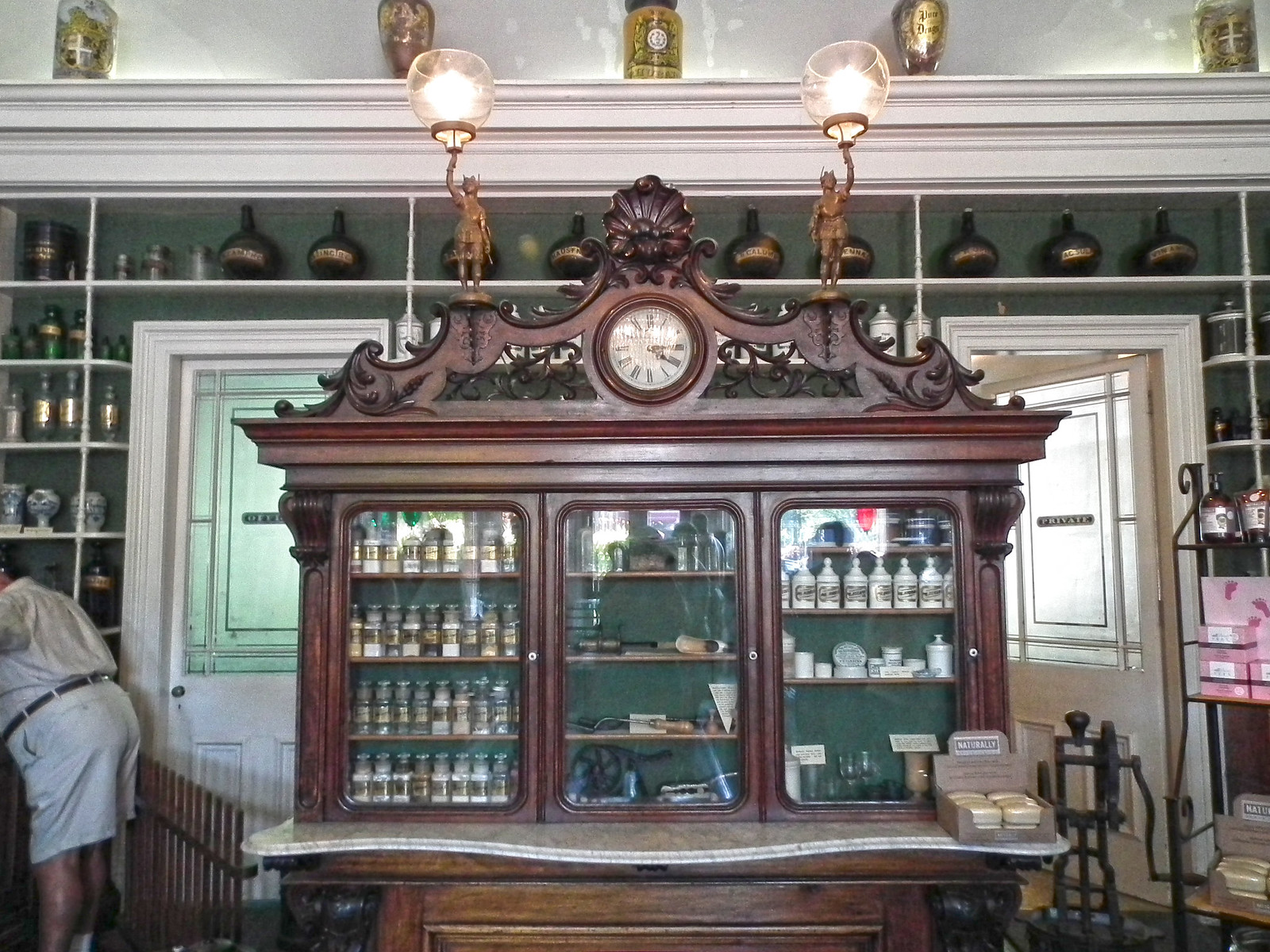This photograph showcases the central feature of an ornate, antique wooden armoire with a rich cherry wood finish, standing out prominently against a forest green background. At the top of the armoire, a clock with Roman numerals is flanked by two gold statues of women holding lamps. The armoire consists of three glass doors on the upper section, which are closed and reveal organized shelves filled with various items: spices on the left, kitchen tools like a pie cutter in the middle, and canisters possibly containing sugar or tea on the right. Below, there appear to be wooden drawers and a flat desk-like panel. To the right side of the armoire, a man in a white shirt and shorts is leaning and looking at something off-camera. The background includes two white doors with glass upper halves, marked "Private," one on each side of the armoire. Additional shelving filled with bottles of various shapes and sizes is also visible, contributing to the store's organized and detailed ambiance.